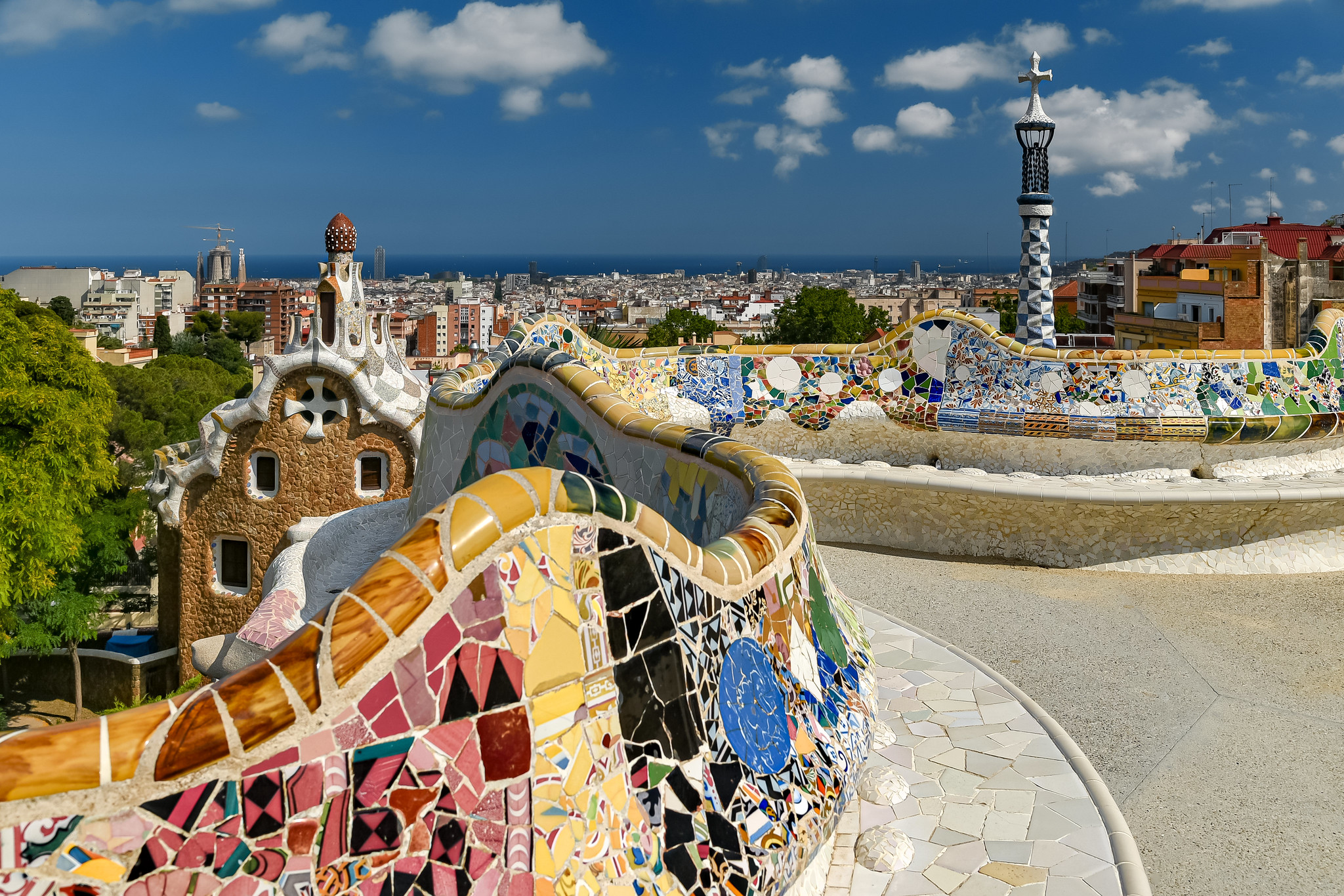The image appears to depict an enchanting scene, possibly from a renowned tourist attraction like Disney World or perhaps a scenic spot in Barcelona. The focal point is the vibrant, winding mosaic wall that runs from the bottom left to the center, curving gracefully before extending to the right. This intricately designed wall features an array of colorful, abstract patterns and shapes, including circles, squares, diamonds, and various asymmetrical forms, all in vivid hues of pink, yellow, blue, and more. The ornate mosaic continues in the foreground, covering the light-colored tile sidewalk and larger square tiles making up the street.

In the background, a picturesque cityscape unfolds, composed of uniquely shaped buildings that exhibit a palette of bright colors. Notably, there are tower-like structures; one to the right bears a white cross atop, possibly signifying a church, and another to the left ends in a brown structure that is a bit indistinct. There is a prominent brown building in the foreground that resembles a gingerbread house, with a cross and a white roof, adding to the whimsical, almost fairy-tale ambiance.

Above, the sky is a clear, crisp blue adorned with cumulus clouds, mostly accumulated to the upper right. The setting, whether a fantastical Disney location or the real charm of Barcelona, bursts with color and artistic design, making it a visually stunning and ornate spectacle.